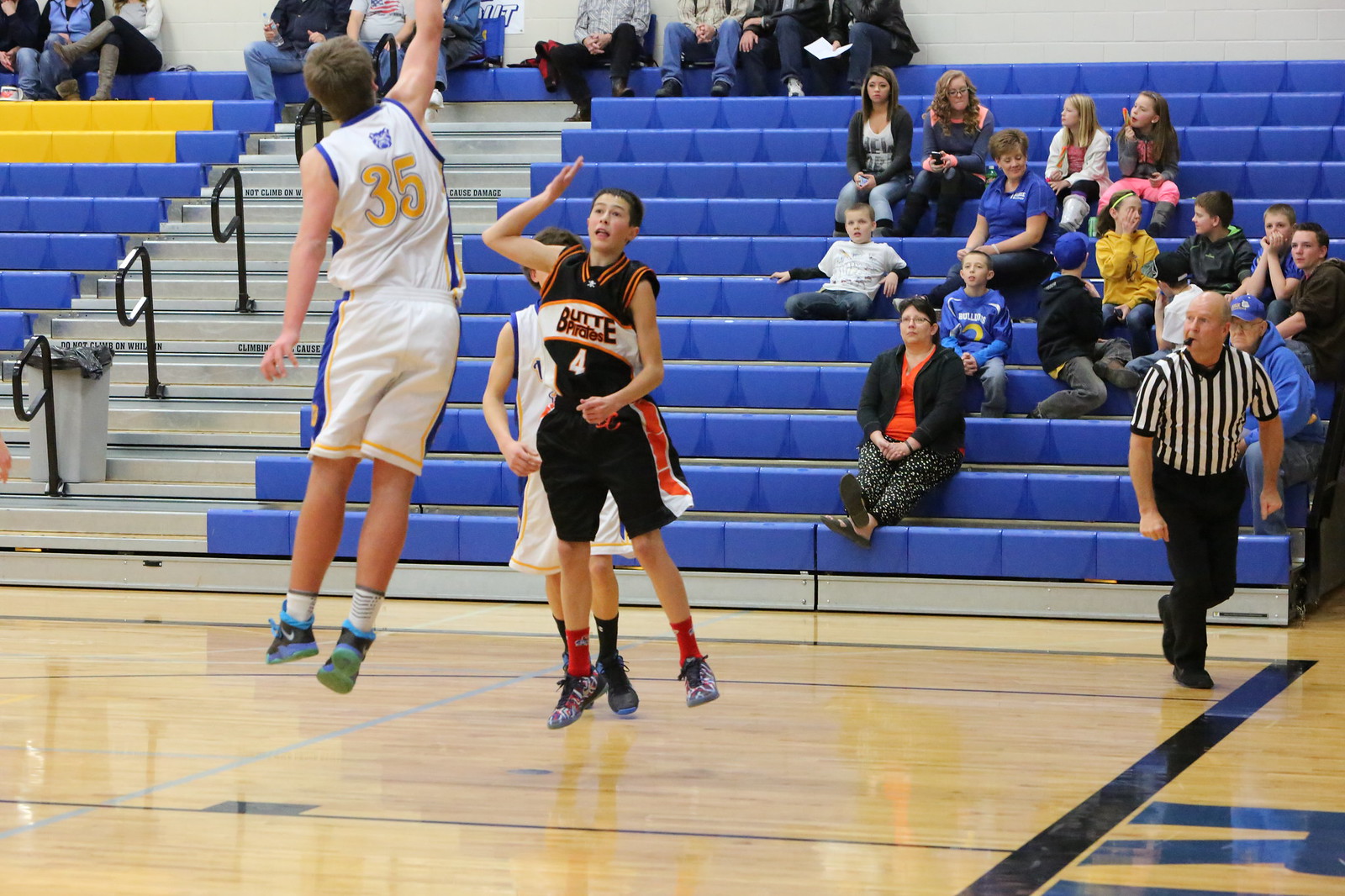This image captures an intense moment of a teenage boys' basketball game. At center court, under the bright indoor gym lighting and on a polished wooden floor, three players vie for the ball. One player wearing a white uniform with blue stripes and the number 35 is leaping into the air with his right arm extended, likely attempting a block. Facing him is an opponent in a black and red uniform, emblazoned with "BUTTE" and the number 4, with his right hand raised defensively near his head and his left arm down. Another player in a similar white uniform is partially obscured by the player in black. To the far right, a referee, identifiable by his striped shirt and holding a whistle in his mouth, is leaning forward with one foot extended back, closely monitoring the play. Surrounding the court, the bleachers are predominantly blue and are filled to moderate capacity, mostly on the right side, with at least twelve spectators. Smaller yellow bleachers are visible on the left, near the top, and a central staircase with gray rails resembling the letter "P" provides access. The gym floor, a light tan color, reflects the indoor lighting, giving the scene a lively and energetic atmosphere.